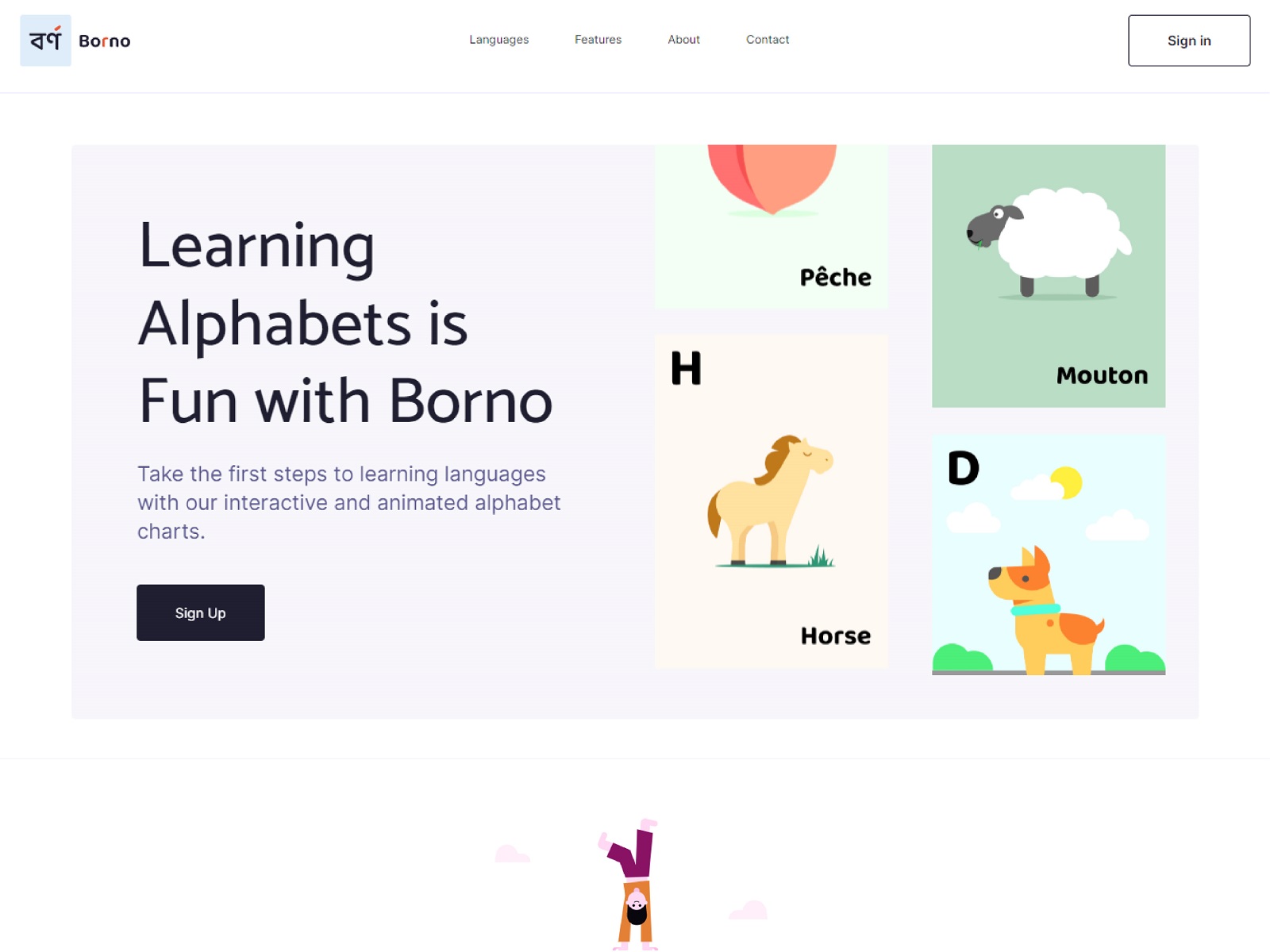The image is a screenshot from a website. In the upper left corner, there is the company name "Borno," with each letter in black font except for the letter "R," which is in gold. Adjacent to the name is a light gray square containing an abstract design resembling a triangle, a right angle, and a circle, which serves as the company logo. The header is white, and centrally located in gray font are the menu options: 'Languages,’ 'Features,’ 'About,’ and 'Contact’. In the upper right corner is a sign-in button, framed with thin black lines.

Prominently displayed in the center of the page against a light gray background is a welcoming message. On the left side in black font, it reads: "Learning alphabets is fun with Borno." Below this, in gray font, it says: "Take the first steps to learning languages with our interactive and animated alphabet charts." Beneath this text is a black rectangular button with "Sign Up" written in white font.

To the right, the page features four cartoonish images in squares. The image in the upper right square depicts a sheep, the one in the lower left square shows a horse, and the lower right square contains a dog.